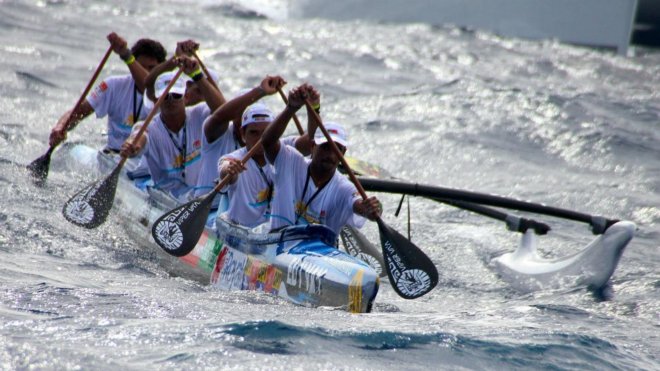In the image, a team of six young male rowers is seen competing in a rowing contest on a turbulent ocean. The team is seated in a slender, outrigger-style canoe, which has two outstretched arms on the right, supporting a small flotation device to keep the canoe upright. The rowers, dressed in white hats, white t-shirts, and sunglasses, paddle with wooden oars that have black paddle ends. The canoe features sponsorship logos and colorful sides, although they are somewhat blurred due to the motion and low resolution of the image. The water around them is rough with waves about one or two feet high, reflecting the sunlight, indicating a very sunny day. The rowers are positioned in a coordinated manner, with three paddling on the left and three on the right side of the canoe. Overall, the setting appears to be a man-made environment created for the competition, despite the naturalistic appearance of the waves and the ocean's expanse in the background.